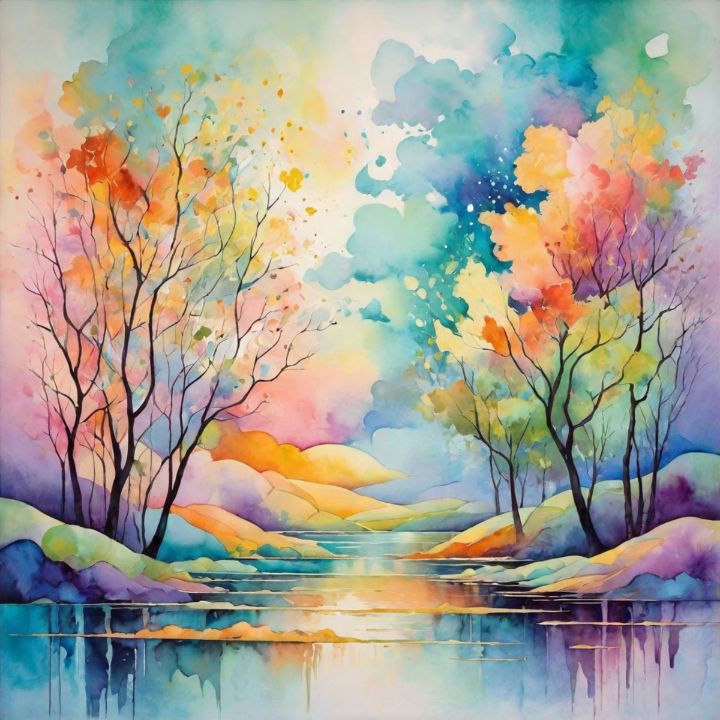The image features a mystical and psychedelic painting, rich in vibrant colors such as blue, red, purple, indigo, orange, and green. The landscape, which resembles a fantasy world, portrays a colorful forest with trees lining a river that flows through hilly terrain. The trees, with black branches and some leaf cover, appear on both the left and right sides of the composition. The center of the painting includes a series of bluish steps, resembling melting ice or snow, adding to the dramatic, surreal quality of the scene. The entire artwork is rendered with a watercolor effect, enhancing its ethereal and dreamlike appearance, despite the absence of any animals or humans. Overall, the painting is a striking and captivating blend of colors and forms, imbuing it with a sense of wonder and beauty.